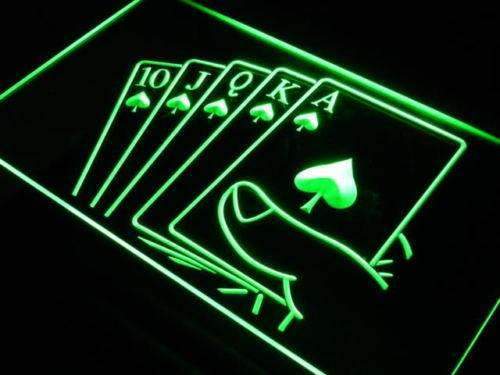This is a detailed and vivid illustration featuring a stylized depiction of a royal flush in spades. The image showcases a hand, though only the thumb is visibly holding the fanned-out cards: the ten, jack, queen, king, and ace of spades. The cards are illuminated with green neon, accented by white highlights, and are set against a completely black background. The entire hand and card composition is enclosed within a large green neon rectangle positioned diagonally from the top left to the bottom right, with the edges of the rectangle cut off, leaving its corners out of view. The cards feature various logos; the ace of spades bears a particularly large green and white logo, while the other cards have smaller logos near their edges. The angle of the image creates a dynamic visual, suggestive of a neon sign one might find outside a casino or gambling parlor, contributing to its vibrant, animated style.